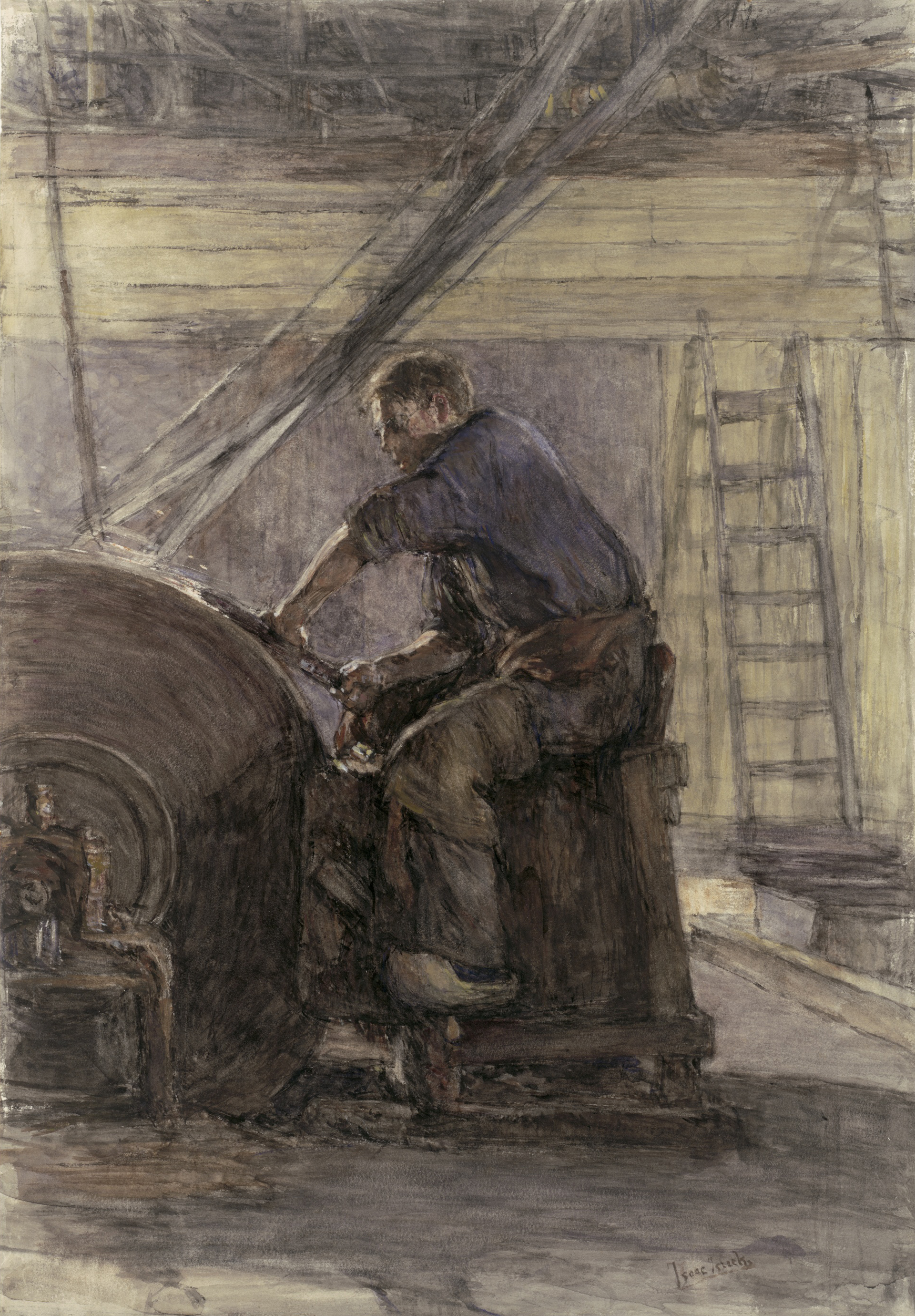The painting depicts a man deeply focused on sharpening a tool against a large, likely pedal-powered, spinning wheel. He sits on a black-colored box, his feet lifted off the bare floor, with one foot poised on the pedal. The man is dressed in brownish pants and a blue shirt with sleeves rolled up, indicative of serious labor. He also has a red sweater tied around his waist. His facial details are not entirely clear, but his brownish hair is discernible. The background features a yellow wall to the right with a ladder propped against it, and a grayish wall to the left, blending into a workshop environment characterized by wooden beams and crossbars on the ceiling. The setting includes several ladders and gives off the impression of a barn or workshop. The artist's signature, somewhat indistinct, is positioned in the lower right corner. The dominant hues in the painting are bluish-gray, brown, tan, and hints of light green.